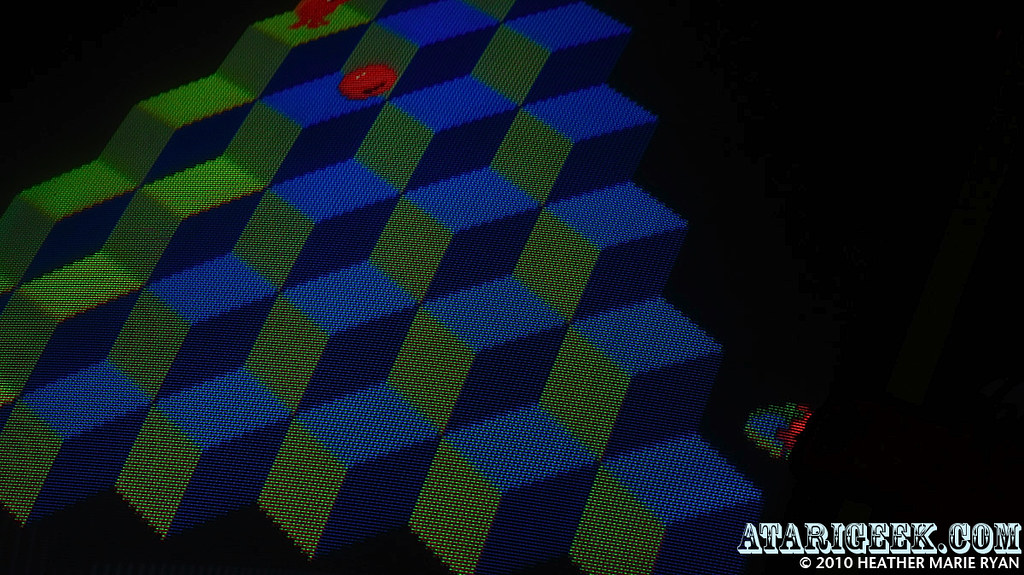This image resembles a retro video game scene with a black background. Squares, colored in green and blue, are stacked on top of each other, increasing in number as they ascend towards the upper left corner. In the bottom right corner, in black and white lettering, is the text "AtariGeek.com, 2010, Heather Marie Ryan." There are several figures in the scene: a small, colorful figure in red, blue, and green located at the bottom right, and two red figures at the top on two of the squares. One of these red figures is round and features a small face. The overall aesthetic evokes a sense of nostalgia for classic video gaming.